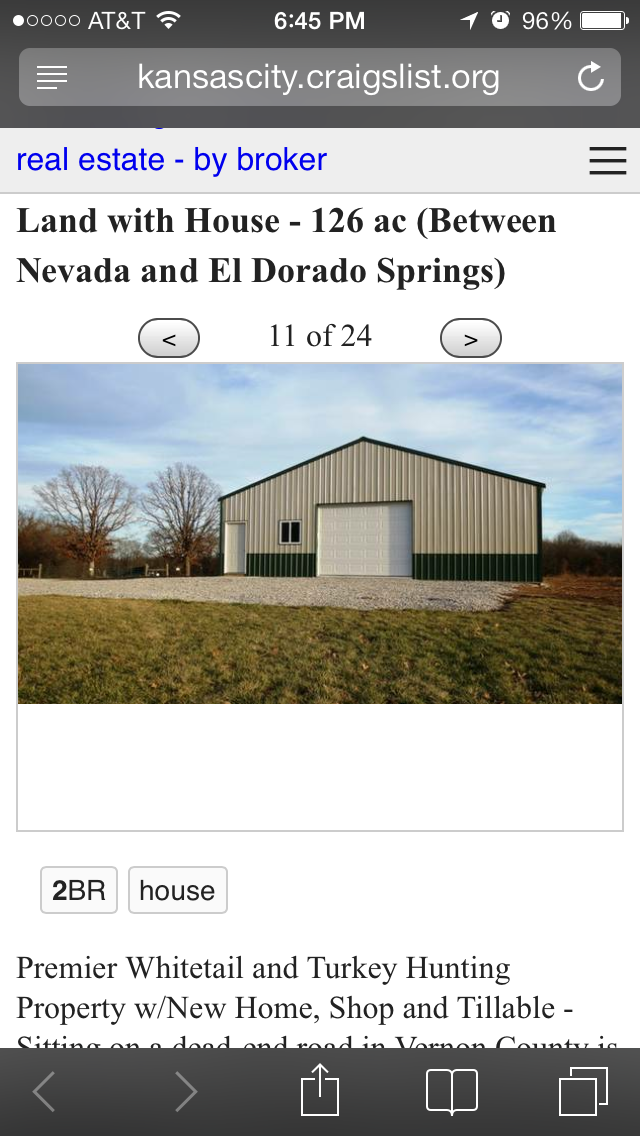The image is a screenshot from a smartphone displaying a Kansas City Craigslist ad in the Real Estate by Broker section. The ad is for a property consisting of 126 acres of land with a house, located between Nevada and El Dorado Springs. The top of the screenshot shows AT&T connectivity with strong signal bars, a time of 6:45 PM, and a battery charged at 96%. The URL is kansascity.craigslist.org, with a gray banner at the top featuring a clockwise arrow symbol.

Below the URL, the text in blue reads "real estate - by broker" followed by "land with house - 126 AC between Nevada and El Dorado Springs" in black text. The listing is indicated as image 11 of 24, with navigation arrows for browsing more images. The prominent photo in the screenshot features a large warehouse or workshop structure, which is half tan and half green, with a large white rolling garage door and a smaller white entry door.

The building has a peaked roof and is set against a backdrop of a blue sky with wispy white clouds and barren trees on the left. The foreground shows a mix of grassy and soil-covered land. Below the photograph, white text on a blank background reads "premier whitetail and turkey hunting property with new home shop and tillable." This suggests the property's appeal for hunting enthusiasts, emphasizing its new home, additional structures, and usable land.

At the bottom of the screenshot, features two labeled buttons: the left button shows "2BR" (two bedrooms), and adjacent to it, a button labeled "house." The truncated line indicates the property is located on a dead-end road in Vernon County.

The bottom of the screen shows smartphone navigation icons, including forward and backward arrows, a share symbol, a pages icon, and a dual-square icon, indicating various operational functions while viewing the ad.